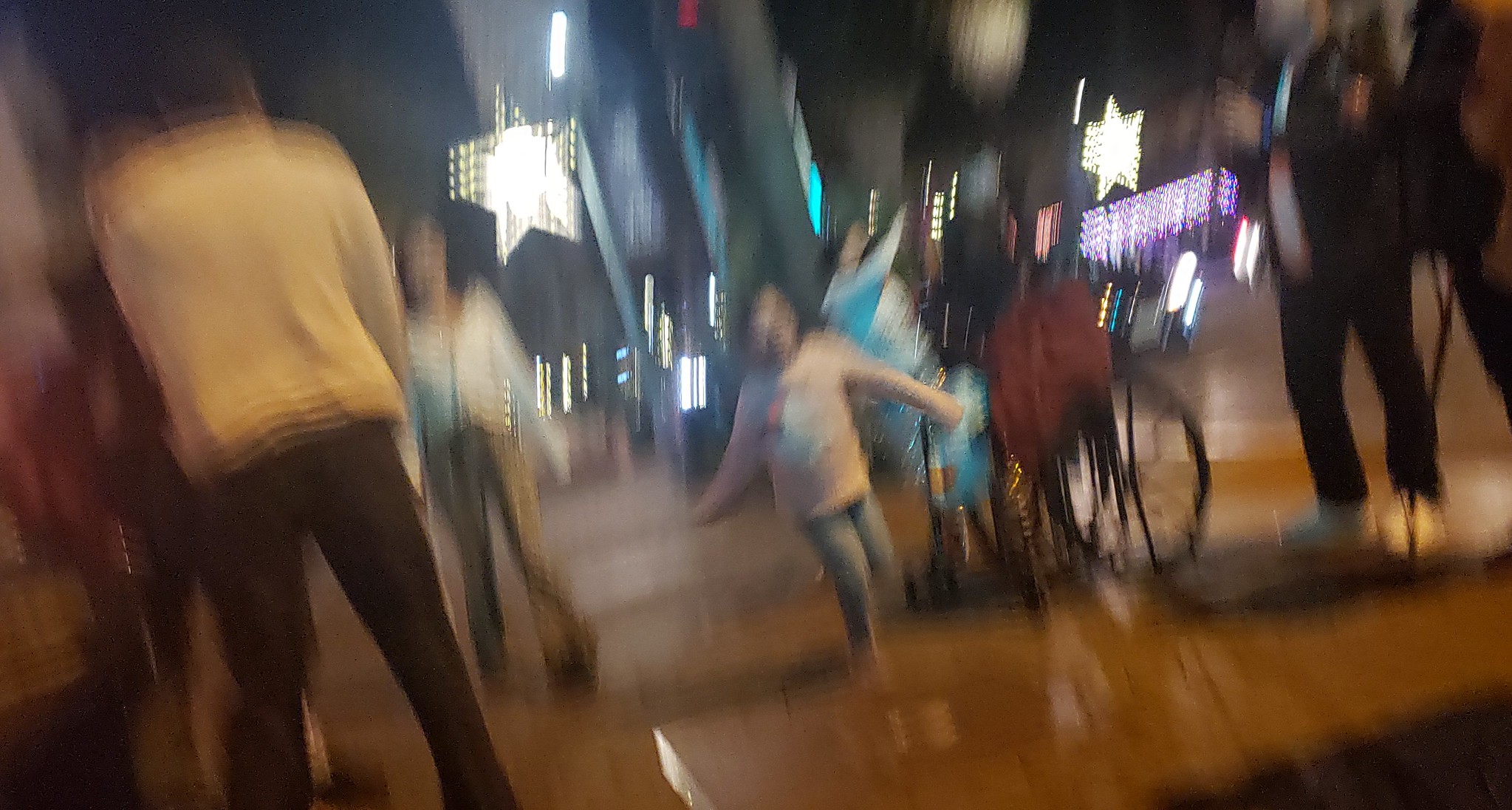This first-person perspective photo captures the energy of a bustling street in motion, evident from the notable blur throughout the image. At its heart is a young girl, joyfully skipping along a polished, shiny brown pavement that suggests a private or semi-private area rather than a public sidewalk. Her outfit—denim jeans paired with a long-sleeved pink woolen jersey—though blurred, stands out vividly.

To her left, a woman can be seen wearing loose, baggy jeans around the ankle, complemented by a white long-sleeved shirt and a sling purse. Ahead of the woman, a man dressed in a similar white long-sleeved shirt and black jeans has his back turned to the camera. The perspective suggests that the camera is at the head level of the skipping child and waist level for the man.

On the right side of the skipping child, there's a hint of a wheelchair or chair, flanked by two individuals who seem to be capturing the moment with their phones held at chest height. In the less distinct background, a prominently blurry yet striking star-shaped LED sign attached to a pole indicates the possible presence of a restaurant or shop. This sign reflects on the right side of the image, hinting at the presence of a mirror or a reflective surface contributing to its duplication in the picture. The overall blur adds to the dynamic essence of the scene, capturing a fleeting glimpse of everyday life in motion.